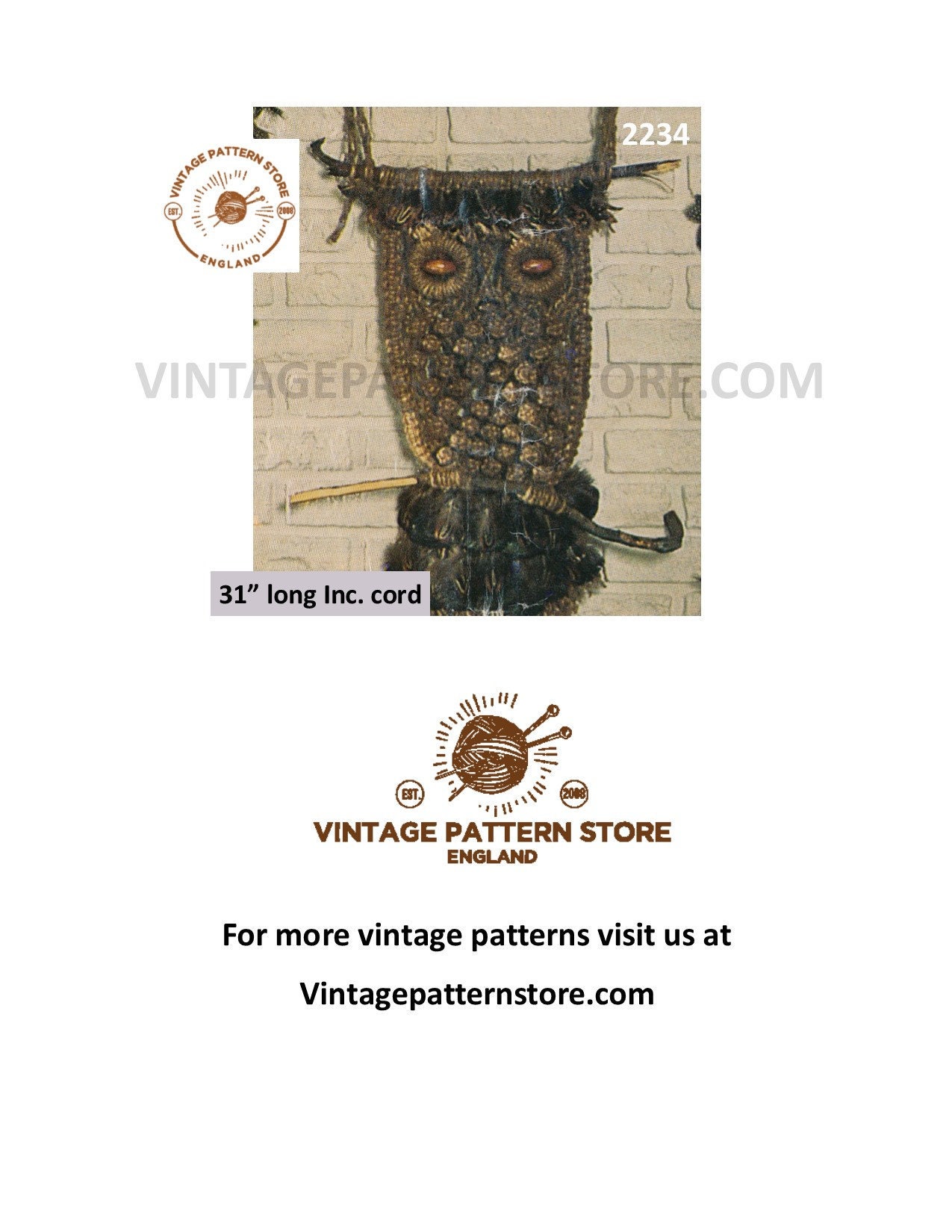The image depicts a photograph of a handcrafted crochet design resembling an owl, positioned against a white brick wall. The crochet creation features two large, circular shapes mimicking owl eyes and a rectangle pattern wrapped around two sticks, enhancing the owl-like appearance as if perched on a branch. The owl design appears to have bronze tones with gold flecks. The photograph includes a watermark, "vintagepatternstore.com," with poor contrast. Additionally, a logo of a ball of yarn with needles is visible, accompanied by the text "Vintage Pattern Store, England." The item number "2234" is displayed in the upper right corner in white text, while a black text caption at the bottom reads, "For more vintage patterns, visit us at vintagepatternstore.com." A small label at the bottom mentions "30-inch lawn ink cord." The overall composition suggests a product photo or listing image for the Vintage Pattern Store, emphasizing its vintage-themed crochet patterns.